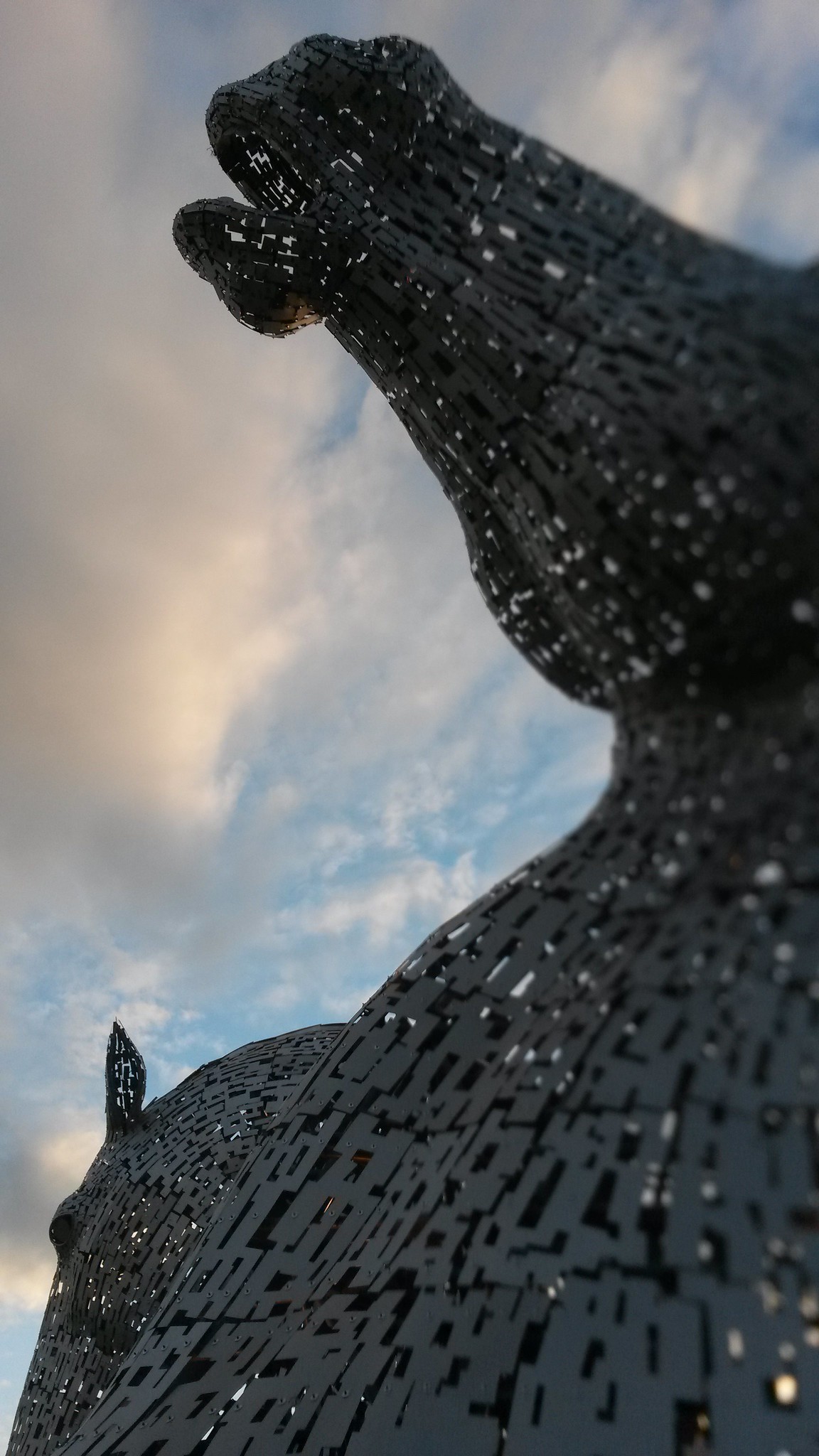This photograph captures a monumental, off-black metallic sculpture viewed from a low angle, emphasizing its immense size against a blue sky filled with puffy white clouds. Constructed from geometrically patterned sheets of metal, the sculpture features a complex design with various shapes, including squares, rectangles, and X-like forms, creating a textured, almost mesh-like appearance with visible gaps. The primary focus of the image is the front portion of a horse's head, including its nose, mouth, and part of its elongated face, protruding into the sky. The left side of the sculpture shows details resembling the horse's eyes and ears, while the right side suggests the neck and chest, possibly with folded wings. The unique artistry of the sculpture gives it a dynamic and open aesthetic, allowing light and sky to filter through its intricate design.